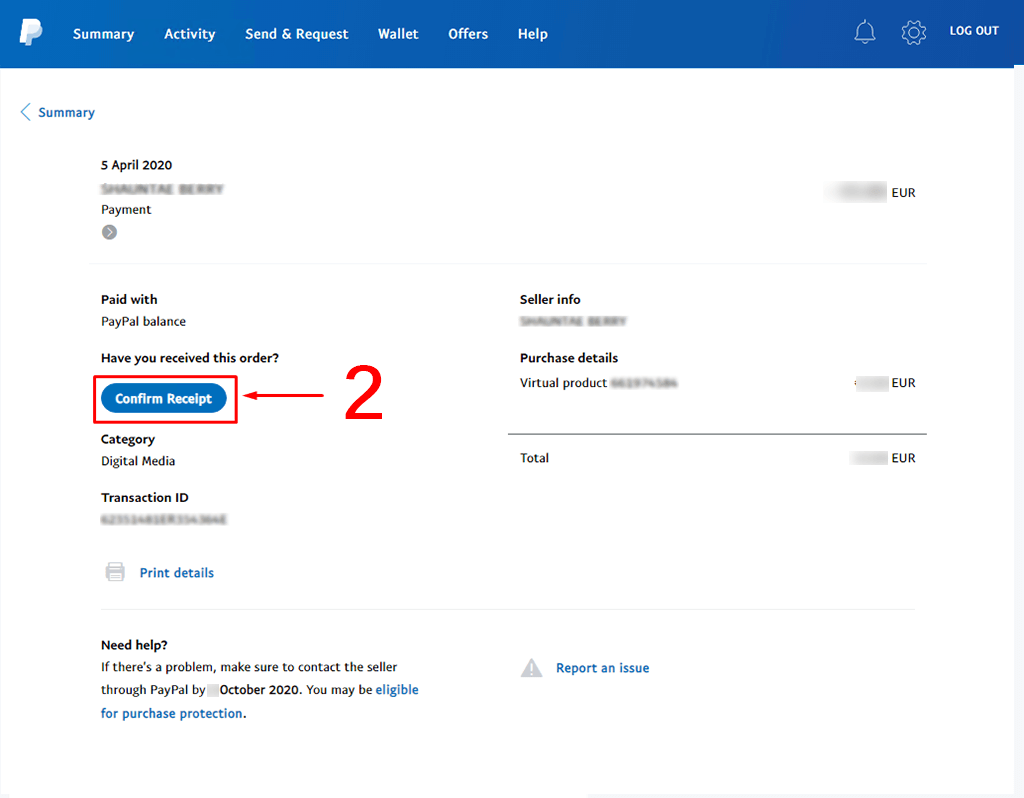This image captures the summary page of a PayPal account as it appeared on April 5th, 2020. The interface displays various navigational elements, including buttons for Activity, Send & Request, Wallet, Offers, Help, and Logout. Central to the page is a detailed transaction overview indicating that a payment was made using the PayPal balance, and there is an inquiry asking whether the user has received their order. 

A prominent blue and white "Confirm Receive" button is highlighted by a red arrow labeled with the number two. Below the confirmation section, the category is marked as "Digital Media," though the specific transaction ID is blurred out. There is an option to print transaction details provided via a link.

Further down, a message offers assistance in case of any issues, advising users to contact the seller through PayPal by October 2020 to potentially be eligible for purchase protection. Another link is present to report an issue.

The seller's information and purchase details are partially obscured, with the seller's name and the total price both blurred out, while the item is identified as a virtual product.